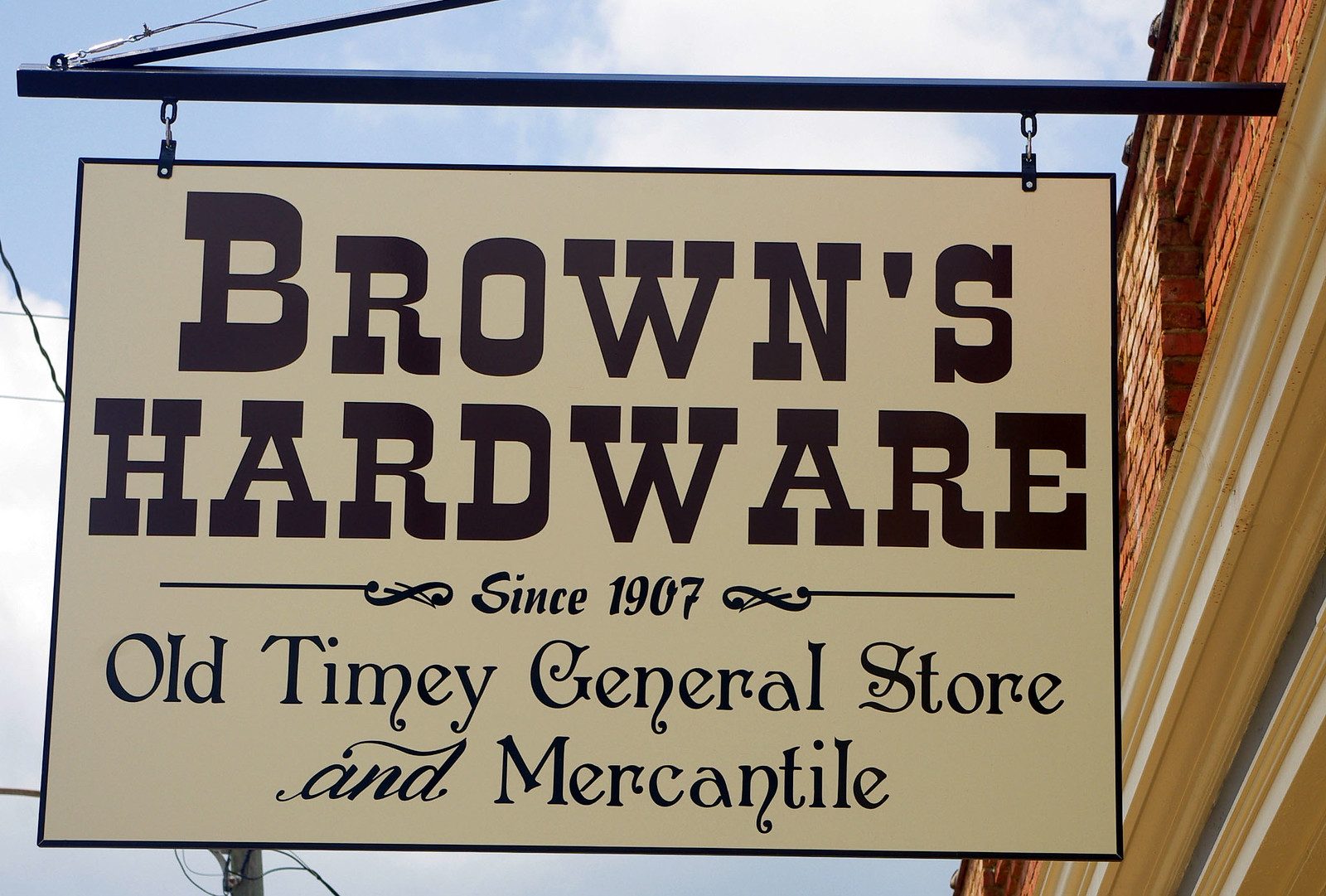The image captures a charming, vintage-style sign for "Brown's Hardware," prominently hung on a black metal bar with chain loops in front of a red brick building with white framing. The tan-colored sign, outlined in black, reads in large dark brown text, "Brown's Hardware," followed by "since 1907" and "old-timey general store and mercantile" in smaller fonts. The sign hangs off to the side of the building amidst a backdrop of a blue sky dotted with white and light gray clouds. There are also some telephone wires visible in the scene as well as a hint of a tree on the left side. The focus of the image is clearly the nostalgic sign, evoking a sense of history and timeless charm.